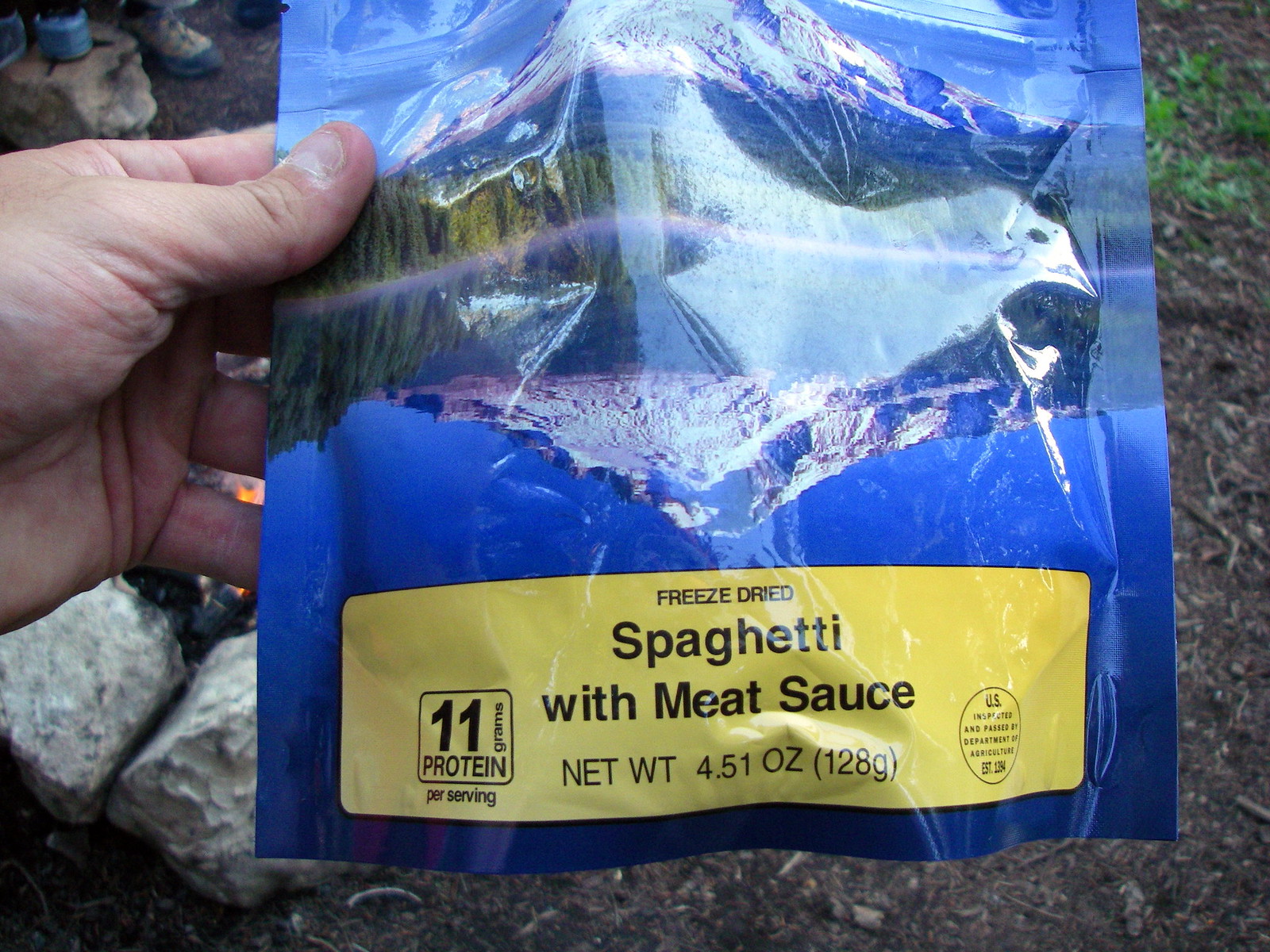A hand from the left side of the image holds a package of freeze-dried spaghetti with meat sauce. The package, prominently blue with a detailed image of mountains, snow, green trees, and water, features a yellow rectangle at the bottom which states “Freeze-Dried Spaghetti with Meat Sauce, Net Weight 4.51 oz (128g), 11 grams protein per serving”. It also has a stamp indicating it has been inspected by the U.S. The photograph is taken outdoors on a grassy patch with large gray rocks visible on the left, indicative of a campsite setting. In the background, you can spot a campfire enclosed by stones, and a boot and part of a pant leg hinting that someone is seated, likely preparing for their meal. This meal, suited for camping, is designed for convenience and outdoor use.